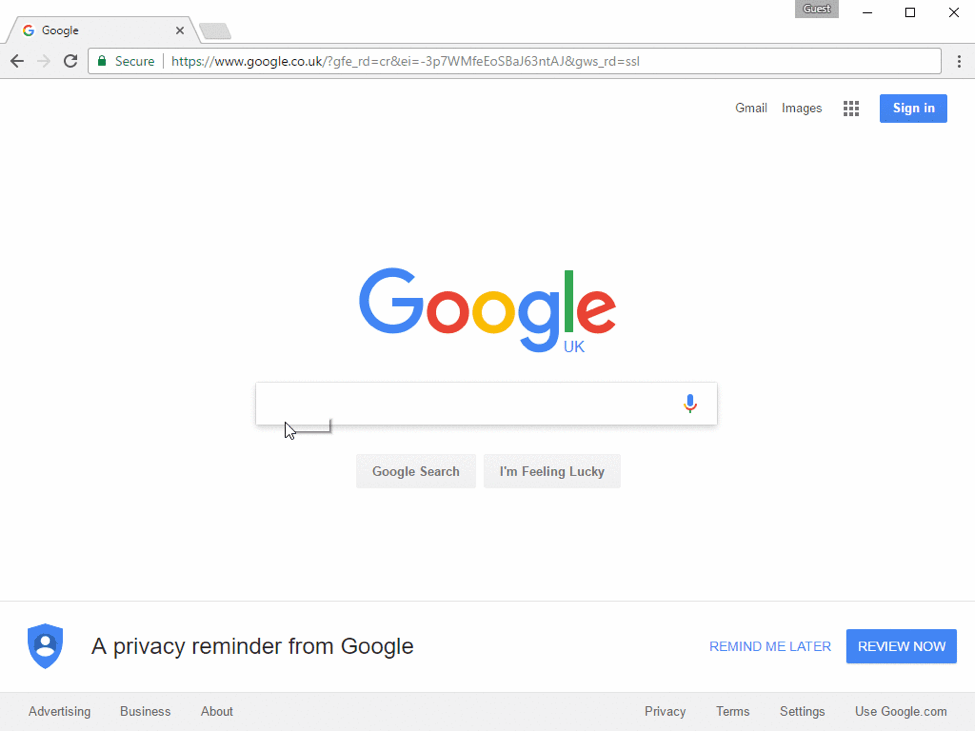The image depicts a screenshot of a web browser opened to the Google homepage. On the top left corner of the browser tab, there is a small, white circle containing the multicolored Google "G" logo, consisting of red, yellow, green, and blue hues. Next to the logo, the word "Google" is written in black font.

Moving to the right side of the tab, there is a gray "X" icon used to close the tab, followed by a gray parallelogram, and then a gray rectangle. Inside this rectangle, the word "Guess" is written in white. Adjacent to this on the very right of the tab are a black dash, a black-outlined box, and a black "X" which are common browser buttons for minimizing, maximizing, and closing the window.

Below the tab bar on the left side of the screen, there's a gray arrow pointing left, a transparent gray line pointing right, and another gray refresh arrow. Following these icons is the address bar, where a green lock icon indicates a secure connection alongside the text "HTTPS" in green. This is followed by "://www.google.com.co.uk" in black text, directing to the Google UK homepage along with additional letters and numbers in the URL for specificity.

On the far right side of the bar, "Gmail" and "Images" are listed in black text. Next to these is a grid of nine black squares, which is a Google apps icon, and a blue "Sign In" button written in white.

The main content area of the browser displays the centered Google logo with "UK" in blue beside it. Just below, there's a large, white search box outlined in gray. Within the search box, a white mouse pointer outlined in black is positioned at the beginning of the text input field. To the right end of this box is a blue microphone icon. Below the search box are two gray buttons; the first one is labeled "Google Search" and the second one reads "I'm Feeling Lucky".